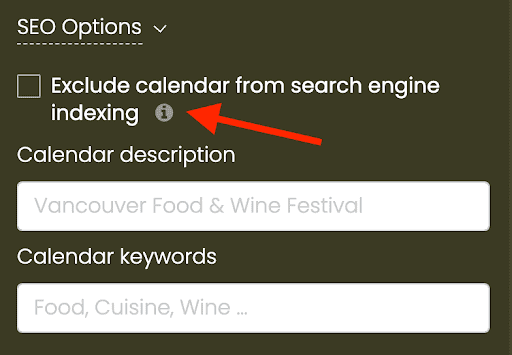The image depicts a panel of Search Engine Optimization (SEO) settings for a calendar feature on a website. At the forefront, there’s a gray circle with an “i” in the center, indicative of an information icon. A prominent red arrow points to a checkbox option labeled "Exclude calendar from search engine indexing," which is currently unchecked, emphasizing the potential to prevent the calendar from appearing in search engine results.

Below this primary option, the interface features editable fields. The "Calendar Description" bar contains a placeholder text, "Vancouver Food and Wine Festival," presented in light gray. Following this is the "Calendar Keywords" section, listing sample keywords including "food," "cuisine," and "wine," suggesting associations with the event. An ellipsis punctuates the keywords, indicating the possibility of adding more terms.

The background of the image has a predominantly gray color with subtle hints of brown and black, contributing to a somewhat pixelated appearance. Despite the graininess, the overall visual focuses on SEO settings, specifically highlighting the option to exclude the calendar from search engine indexing. The interface is part of a website's SEO configuration tools, offering a glimpse into detailed SEO management options for events.